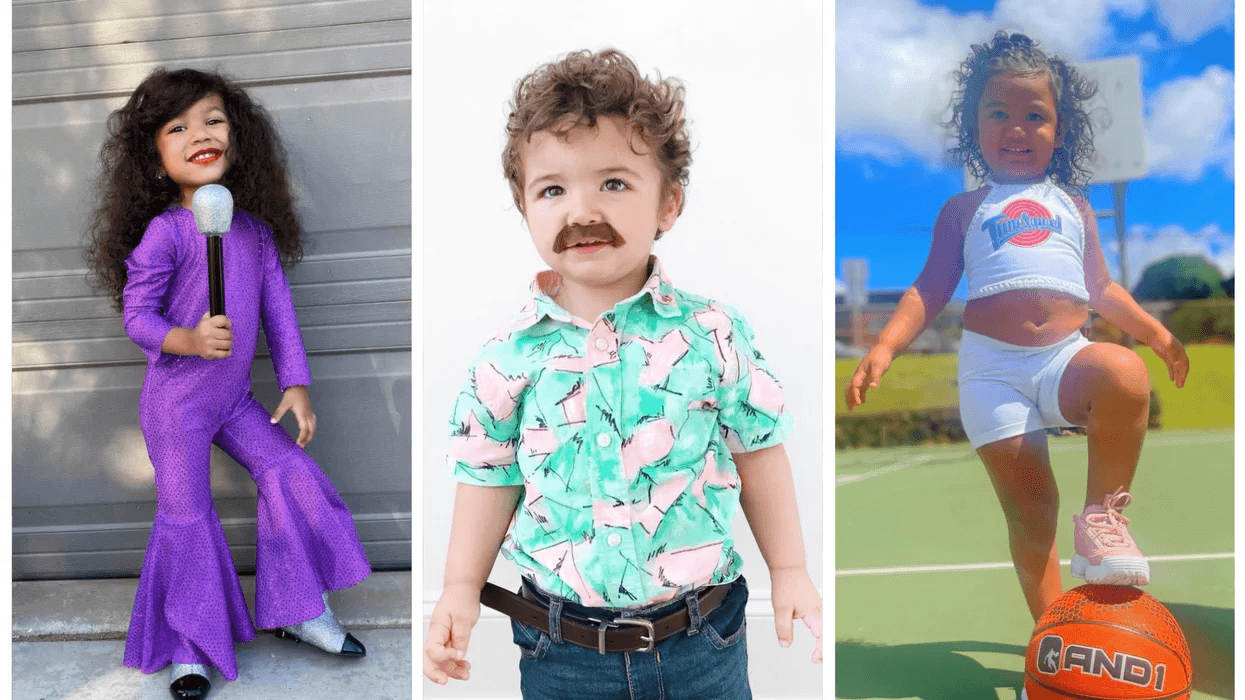The image is a composite of three young kids, each dressed in distinctive outfits, likely for a costume event. On the left, there is a smiling girl with long, curly brown hair wearing a purple sparkly jumpsuit with wide, flared legs. She sports red lipstick and holds a black microphone with a sparkling head, appearing as if she's a pop singer. In the center, a boy with tousled brown hair has a painted mustache and wears a vividly patterned green and pink shirt. He completes his look with blue jeans and a brown belt that hangs loosely, suggesting it’s too large for him. Lastly, the rightmost panel features a girl standing confidently with one foot resting on a basketball labeled "And1." She has curly brown hair and wears a white crop top and white shorts. Her outfit and stance, complete with pink and white sneakers, evoke an image of an athlete, possibly inspired by Space Jam's "Tune Squad." She's positioned on a basketball court, adding to the sporty theme.